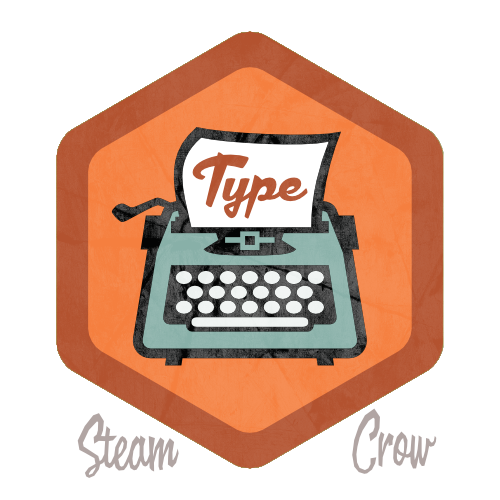The image features a central hexagonal figure with a dark orange, almost reddish border and an orange interior. Positioned centrally within this hexagon is a stylized drawing of an old-fashioned, light green typewriter. The typewriter has white keys and a white space bar, emphasizing its vintage charm. A piece of paper emerges from the typewriter, bearing the word "TYPE" in orange cursive text. At the bottom corners of the hexagon, the word "STEAM" appears in gray cursive on the left, while "CROW" is inscribed in gray cursive on the right. The typewriter and the piece of paper both feature bold, black outlines to make them stand out prominently against the background. Encapsulating all these elements, the overall backdrop of the image is white. The image gives the impression of being a patch, badge, or perhaps a logo, possibly associated with someone's steam account or a similar platform.